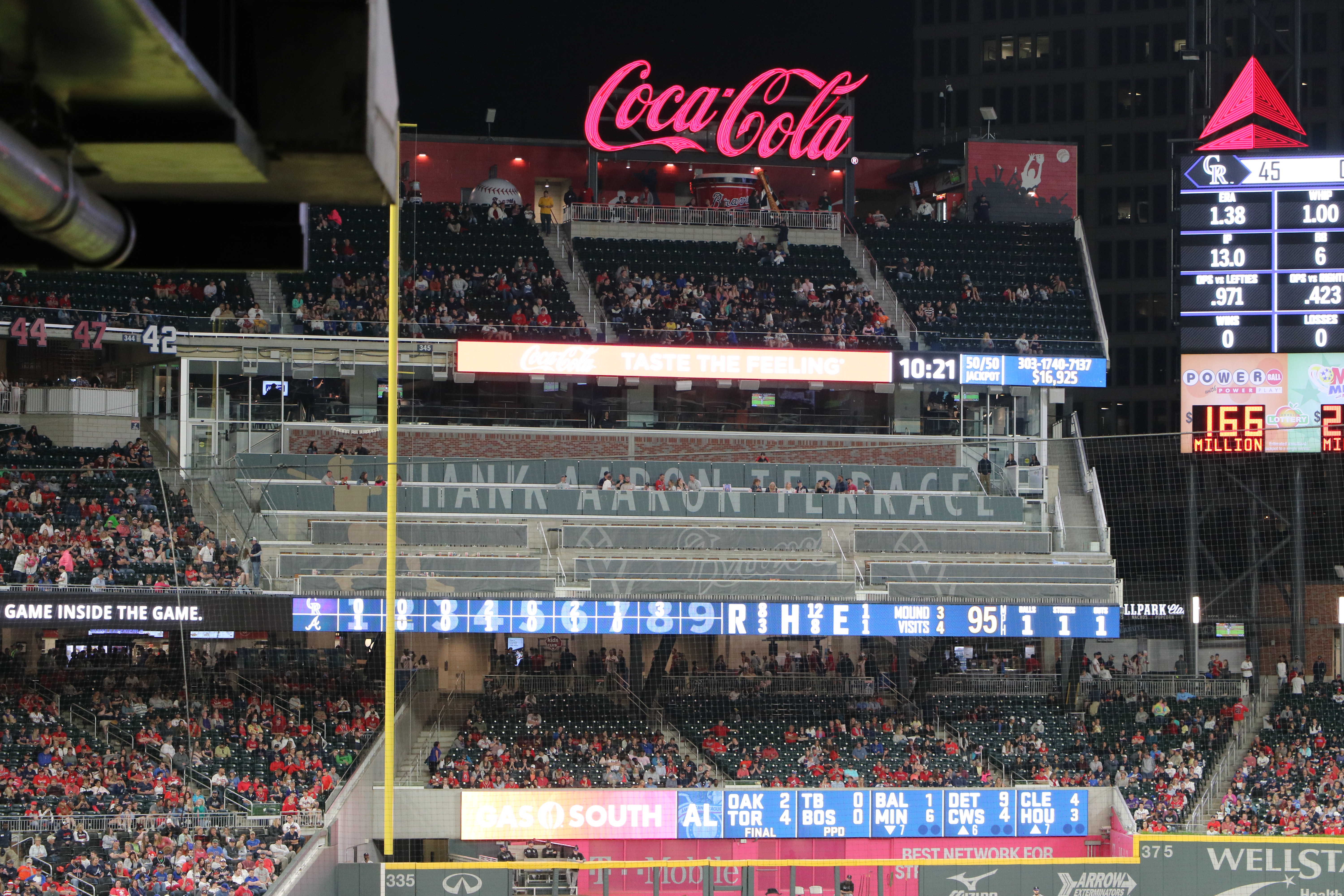This image features a multi-tiered baseball stadium bustling with activity. The bottom row of bleachers is mostly filled with spectators, while the middle tier is more sparsely populated and the top row is about a quarter full. Dominating the scene at the top of the grandstands is a red, illuminated Coca-Cola sign, under which reads “Hank Aaron Terrace.” Spectators are seen in a variety of colors, although red t-shirts are particularly abundant. On the right side, above a detailed scoreboard, a bank logo catches the eye. The scoreboard displays various player statistics and game scores, including Oak 2, TOR 4, Ball 1, MIN 6, Detroit 9, CWS 4, Cleveland 4, Houston 3. Blue backgrounds with numbers and letters adorn the front of the grandstands, adding to the vibrant visual tapestry. Text reading “Game inside the game” is scattered around the venue, enhancing the immersive sports experience.